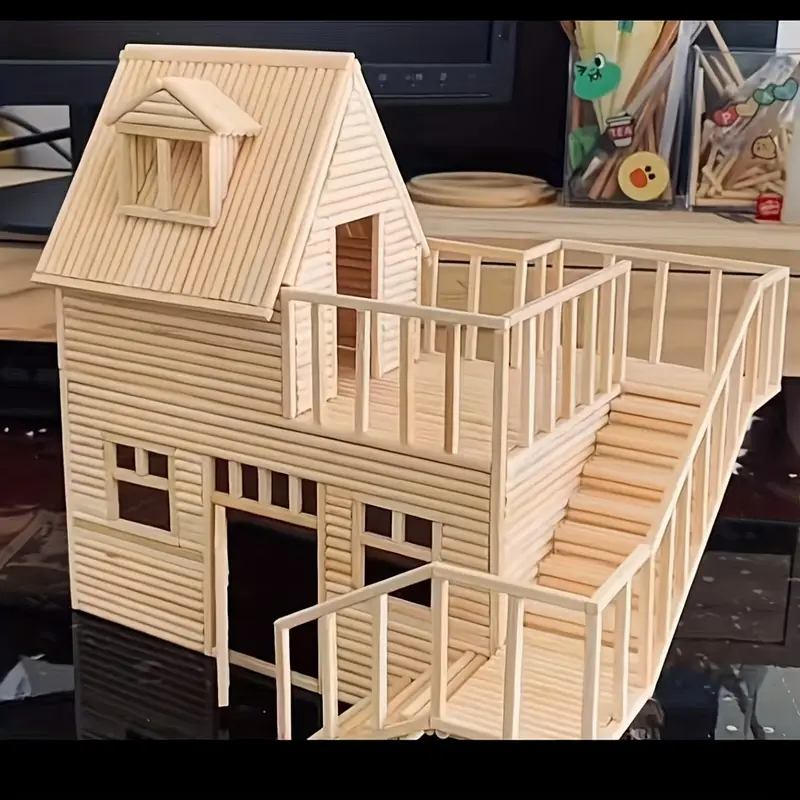This photograph depicts a detailed model of a two-story wooden log cabin, constructed from light-colored wood pieces reminiscent of miniature logs or popsicle sticks. Dominating the front of the model is a large door with four small windows above it, flanked by two windows on either side. On the right side of the building, a staircase ascends to a deck on the second floor, which extends around the building and provides access to a door situated under a triangular gabled roof. In the background, the scene contains model-making tools and supplies, including clear containers adorned with stickers of a green frog, a yellow duck, and hearts. Additionally, the background features a mahogany shelving unit with various items, including match-like sticks and pens in a lucite box.